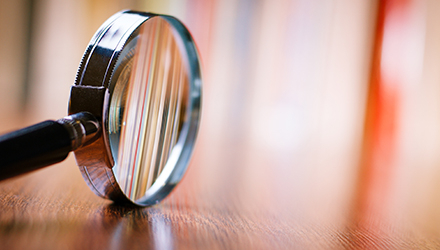The image depicts a magnifying glass positioned slightly to the left of center on what appears to be a blurred wooden surface. The magnifying glass has a shiny silver trim and a black handle that extends out of the image frame to the left. It is balanced on its side, supported by both the edge of the glass and the handle. The background is heavily blurred but features strips of red, blue, and a lot of light pink, with some hints of white and black. These colorful stripes are also reflected in the glass of the magnifying glass, adding a dynamic touch to the overall composition. The wood surface underneath has a shiny wood grain that is mirrored on the glass. There are no people or writing in the image, just the magnifying glass and the blurred, colorful background.